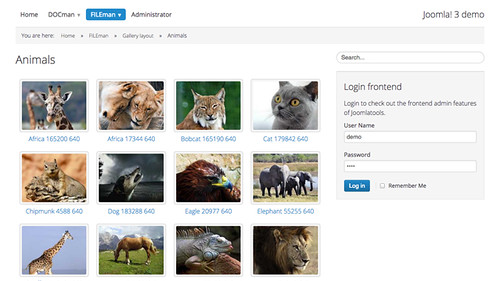The image displays a computer screen with a white background. At the top left, several navigational elements are listed in black text, starting with "HOME" followed by "DOCMAN." Adjacent to these, there is a section with a blue background featuring white text that reads "FILEMAN." Continuing right from this, the text reverts to black, stating "administrator." To the far right, the sequence includes "JOOMIAL" and "free demo."

Beneath these labels, a horizontal gray line separates the navigation from the content below. Under the line, it reads "YOU ARE HERE," followed by the category "ANIMALS."

The main content area showcases various animal images. The first image is of a giraffe, followed by a picture of a gray cat with a startled expression. Subsequent images include elephants.

To the right of these animal pictures, there is a sidebar with a light gray background. It features sections labeled "LOGIN" and "FRONTEND," along with an invitation to "LOGIN to check out the frontend admin features."

The bottom right corner of the image remains a blank white space.